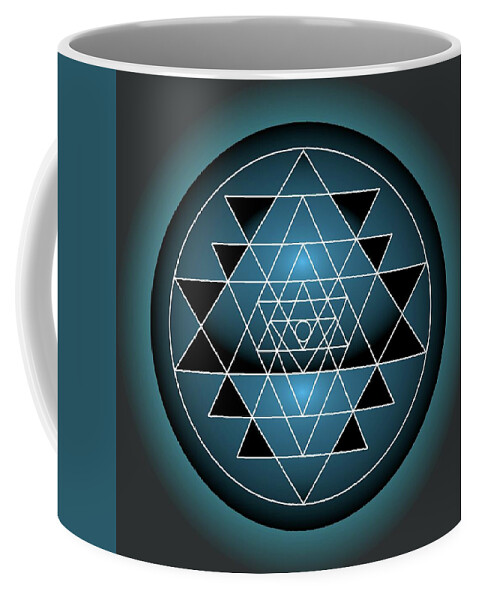This composite rendering presents a white mug set against an entirely plain white background, lacking any shadows. The mug's handle is displayed subtly on the left side. Adorning the mug is a complex, geometric design. The main image on the mug features a black background with a large dark turquoise strip on the left. Centrally, a black rectangle houses an intricate design. This central pattern includes a black circle surrounded by a thin white outline and numerous intersecting triangles creating a multi-layered, step-like pattern that resembles traditional Native American or indigenous art. The triangles, drawn with white outlines, vary in size, forming smaller black-shaded triangles where they overlap. At the very core of this elaborate design, a tiny circle can be found. The colors include dark turquoise and various shades of black and blue, emphasizing the geometric and somewhat mystical aesthetic.